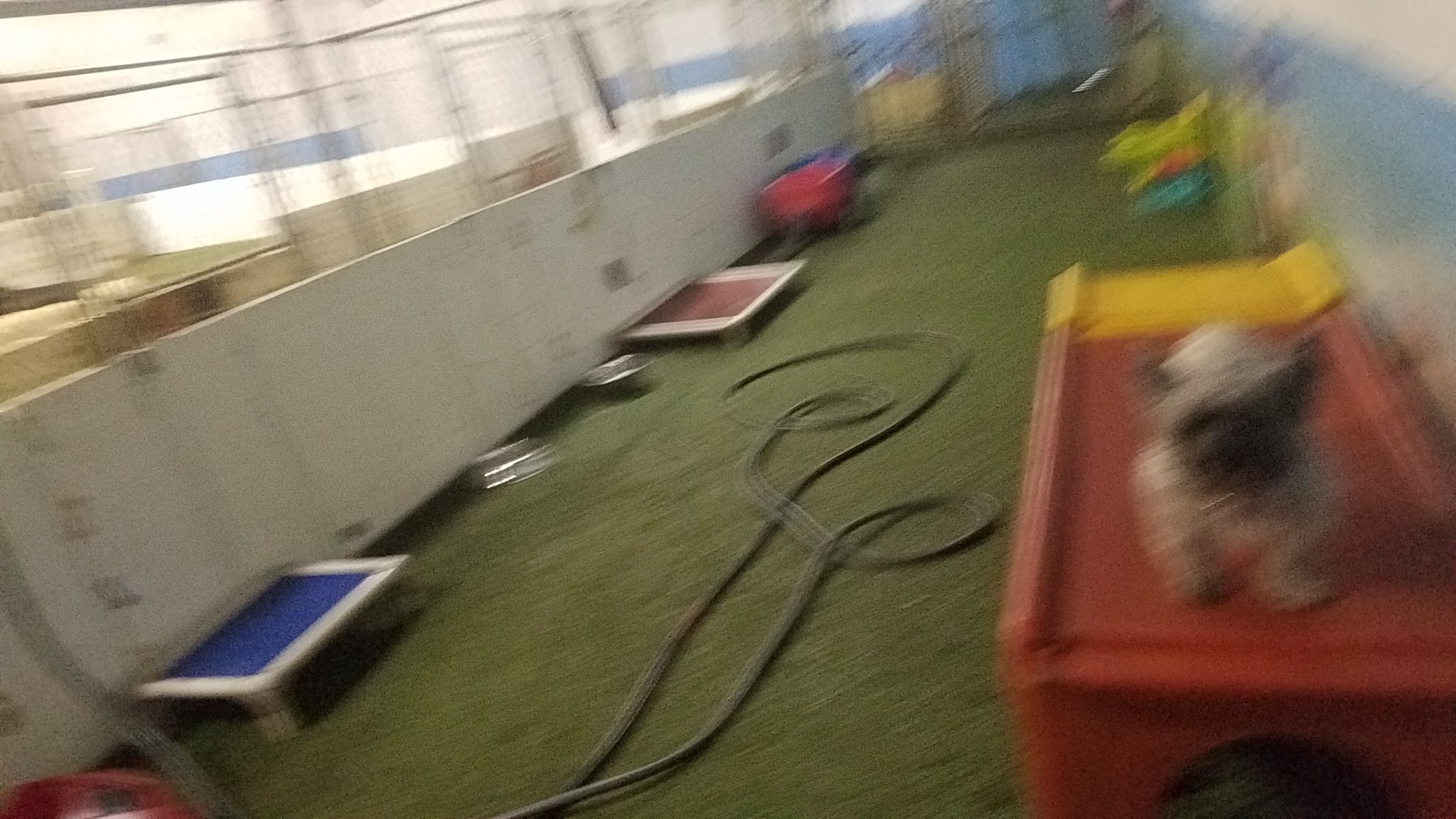This blurry and grainy photograph captures the inside of a large facility, likely designed for animals. The ground is covered in dark green synthetic turf, giving the appearance of an animal-friendly environment. In the center-right of the image, there is a raised maroon-red plastic desk, accented with yellow at the back, on which a small, short-statured dog with tan fur, dark chocolate brown ears, and a similarly colored face is perched.

Along the floor of the facility, a dark green hose is visible, although its ends extend out of the frame. To the left, there are small, raised platforms resembling trampolines. One of these platforms has a blue interior and white exterior, while another features a white border with a red interior. Between these platforms, two silver dog bowls are placed.

Further to the right, objects including a red wagon and a dark blue item blur together. On the left side of the image, what appear to be kennels are arranged at an angle. These kennels have white doors that reach halfway up and are topped with chain-link fencing, suggesting secure enclosures for the animals. The back of the image fades into a mix of greens, blues, whites, and reds, creating a blended, unfocused backdrop. The white walls and ceiling, coupled with a strip of dark blue on the far right wall, complete the setting of this animal care facility.